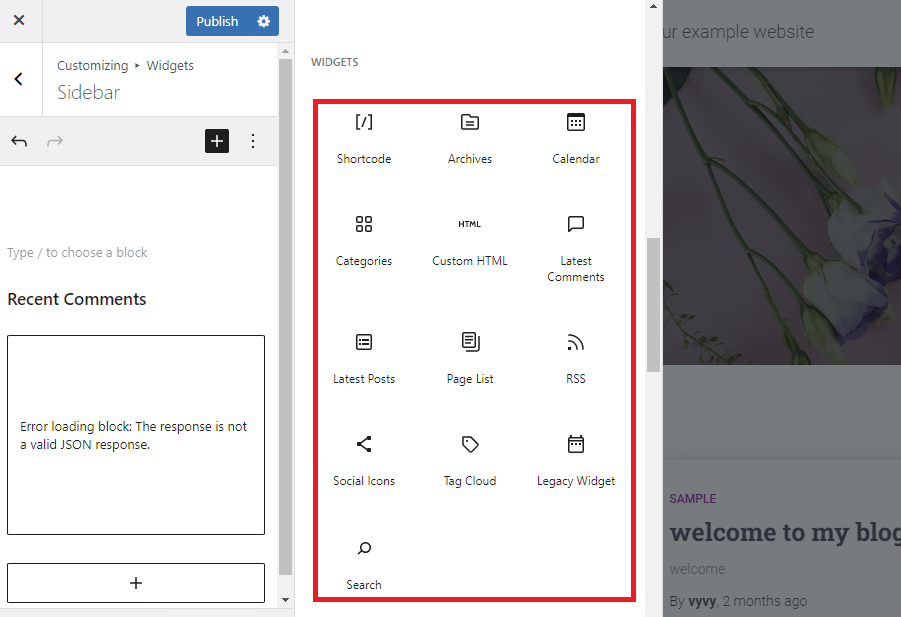**Screenshot Description: Widget Configuration Interface**

The screenshot depicts a widget configuration interface within a website customization tool. 

**Detailed Breakdown:**

1. **Central Focus:** 
   - **Highlighted Section:** The central part of the screenshot is distinctly marked with a red border, emphasizing the main area of interest. 
   - **Background:** The section has a white background and features the word "widgets" in very small letters at the center. 

2. **Widget Layout:**
   - The highlighted area is organized into five rows and three columns of widgets.
     - **First Row:** 
       - Widget Titles: Shortcode, Archives, Calendar.
     - **Second Row:** 
       - Widget Titles: Categories, Custom HTML, Latest Comments.
     - **Third Row:** 
       - Widget Titles: Latest Posts, Page List, RSS.
     - **Fourth Row:** 
       - Widget Titles: Social Icons, Tag Cloud, Legacy Widget.
     - **Fifth Row (Bottom Left):**
       - Widget Title: Search.

3. **Sidebar and Customization:**
   - **Upper Left Corner:** Displays a publication bar labeled "Customizing: Widgets - Sidebar".
   - **Error Message:** Below this bar, an error message reads, "Recent Comments: Error loading block: The response is not a valid JSON response."
   - **Interaction Buttons:** There is a plus button (+) indicating the option to add a new block.

4. **Additional Interface Elements:**
   - **Upper Right Corner:** Indicates the presence of an example website view.
   - **Bottom:** A footer message reads, "Welcome to my blog", which might be part of the mockup or demonstration website shown in the screenshot.

This detailed screenshot highlights the process of adding and organizing widgets while customizing a website's sidebar, providing users with a visual guide through the widget configuration interface.